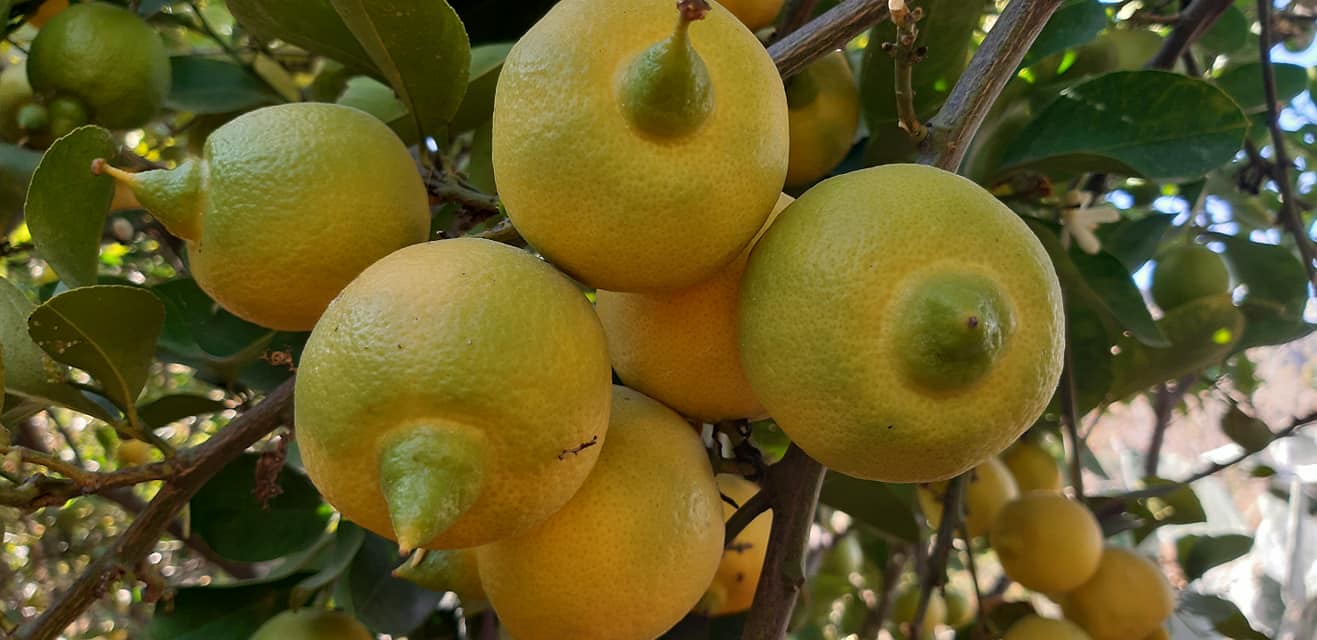This close-up photograph captures a vibrant citrus tree adorned with ripening fruit. The tree's branches are a rich brown, contrasting with its curling dark green leaves. The citrus fruits, resembling lemons, display a spectrum of maturity: some are fully yellow, some are green, and others exhibit a blending hue. The yellow fruits have a distinct citrus texture with a pointy green end. Highlighting the composition, several fruits sit prominently in the center, while others dapple the background, set against a green canopy with sunlight filtering through. The scene vividly showcases the stages of the citrus fruits' ripening process on this lush tree.